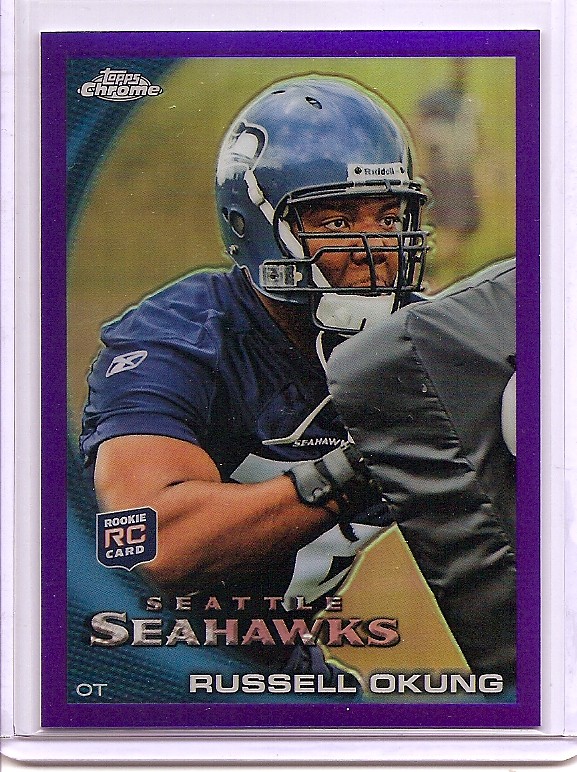The image showcases a collectible football card encased in a protective sleeve, featuring a white outer border and a purple inner border. The top left corner of the card displays the "Topps Chrome" logo with an oval-shaped football icon. At the center of the card is a photograph of Russell Okung, a player from the Seattle Seahawks, dressed in the team's blue helmet with the Seahawks logo and a matching blue jersey. The jersey prominently features his number and he is seen holding a black blocking pad, suggesting a practice scenario. The card is marked with "Rookie RC Card" and a shield icon, in addition to the text "Seattle Seahawks" in pink and "OT Russell Okung."